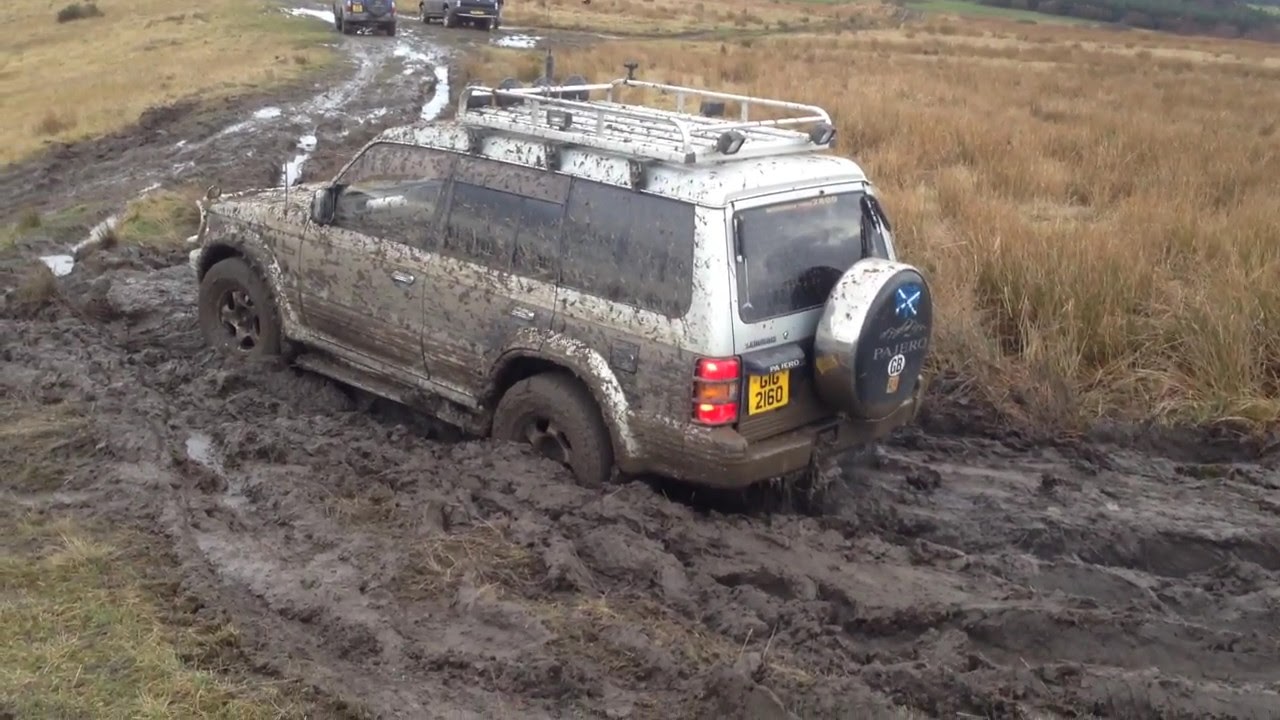The image depicts a silver Jeep, with a license plate featuring "BLB" and "2160" on a yellow background, stuck in a deep, muddy terrain. The left front wheel is only slightly embedded in the mud, while the back left wheel is halfway submerged, hinting at the difficulty of its situation. The Jeep is extensively splattered with thick, brown mud, especially on the sides and roof, which is equipped with a partially mud-covered chrome roof rack. The vehicle's four doors and rear hatchback are barely visible under the layer of mud. A noticeable muddy trail extends from the bottom right corner, curves through the center, and stretches to the top left, blending with the flat terrain. Surrounding the muddy path is a mix of yellowish, dead grass and green brush, highlighting the off-road environment. In the background, two other vehicles are discernible, suggesting they either avoided this treacherous muddy stretch or managed to navigate it successfully. The chaotic muddy scene encapsulates the intensity of the off-roading experience.